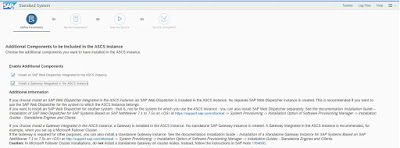A very small and hard-to-read web page focused on SAP technology. The page appears retro in design with a light gray background and predominantly black text. Several subsections are present at the top of the page, though the exact titles are unclear, with the words "additional" and "components" partially visible. The visual style suggests a mature, widely-used business application, likely related to enterprise analytics or management software. Due to the small and unclear text, further details about the specific functionalities of SAP on this page are indiscernible.